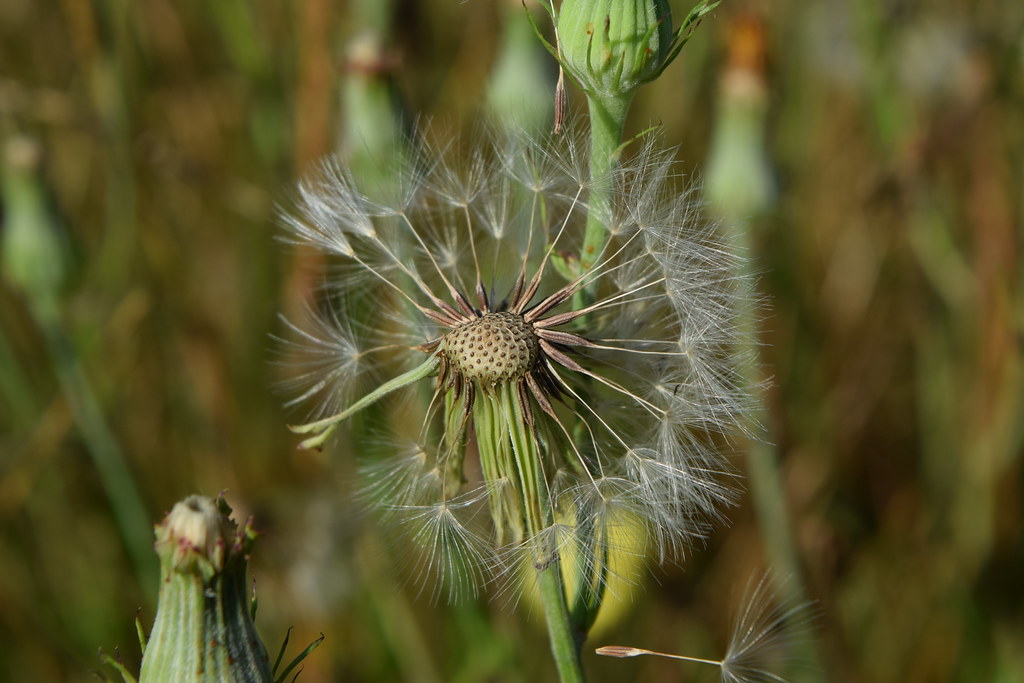The image captures a close-up of a nearly-expired dandelion in sharp focus at the center. The dandelion, with its characteristic wispy white seeds, reveals that many of the seeds have already been blown away, though about 20 remain clinging to the right side of its round head. Surrounding the central dandelion, the blurred background reveals a collection of green stems with unopened buds and additional brown twigs. Notably, in the lower left corner, there's a dandelion bud yet to bloom, exhibiting tightly closed green leaves encasing white petals. The diffuse, dark background, dotted with hints of green foliage and patches of dirt, suggests an outdoor setting on a sunny day, devoid of any visible horizon or sky. The overall scene emphasizes the life cycle of dandelions, from bud to nearly complete seed dispersal, framed against a beautifully blurred natural backdrop.